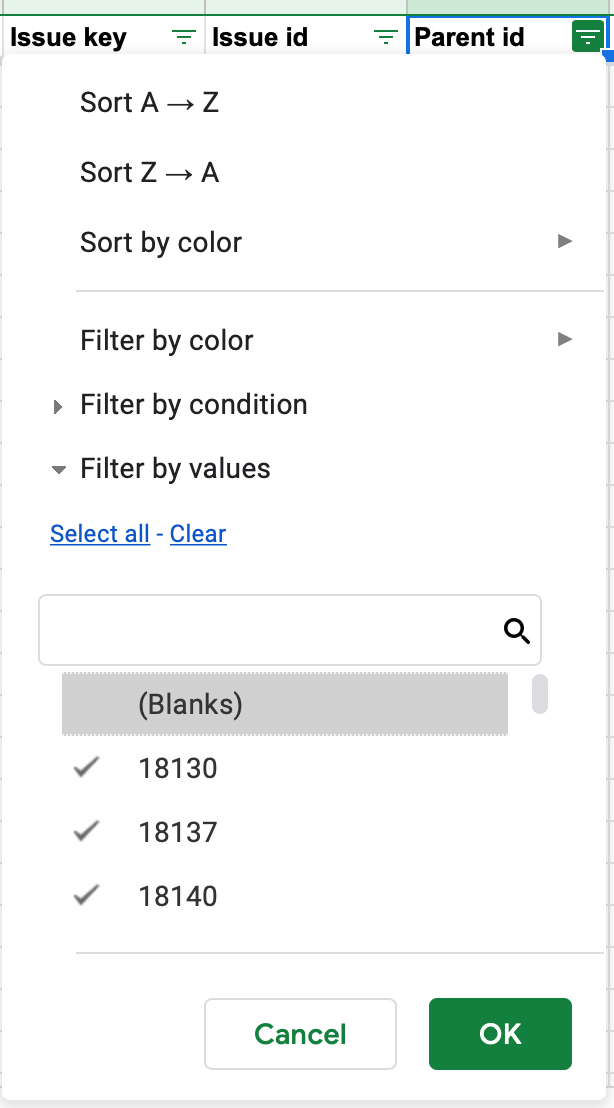**Detailed Caption:**

The image features a software interface for handling issues, displaying several key elements for managing data. At the top, there is an "Issue Key" and an "Issue ID" field, each corresponding with specific identifiers for the issues listed. Adjacent to these is a "Parent ID" field, distinguished by a blue square highlighting it.

To the right of these fields, the interface is adorned with several lines: white lines immediately to the right of the "Parent ID" field, followed by green lines extending further right. 

Sorting options are prominently displayed, including:
- An "A-Z" sorting button.
- A "Z-A" sorting button.
- A "Sort by Color" option represented with an arrow.
- A "Filter by Color" option with another arrow.
- An "Arrow filter by condition."
- A "Down arrow filter by values."

Below these sorting and filtering options, there is a selection area with all options cleared, presented in blue with blue lines under each section, separated by dashes.

For specific issue selections, a chat text field is visible, including a black search icon. A gray square labeled "(Blanks)" in black text is also present. Underneath this gray square, there are gray check marks next to the issue IDs 18130, 18137, and 18140, indicating selected issues.

A gray dividing line separates this section from action buttons at the bottom. The "Cancel" button, highlighted in green, is framed by a gray line and is shaped into a square. Next to it, the "OK" button is featured in white text within a green square.

The interface is designed to offer comprehensive and detailed methods to sort and filter issue data effectively.